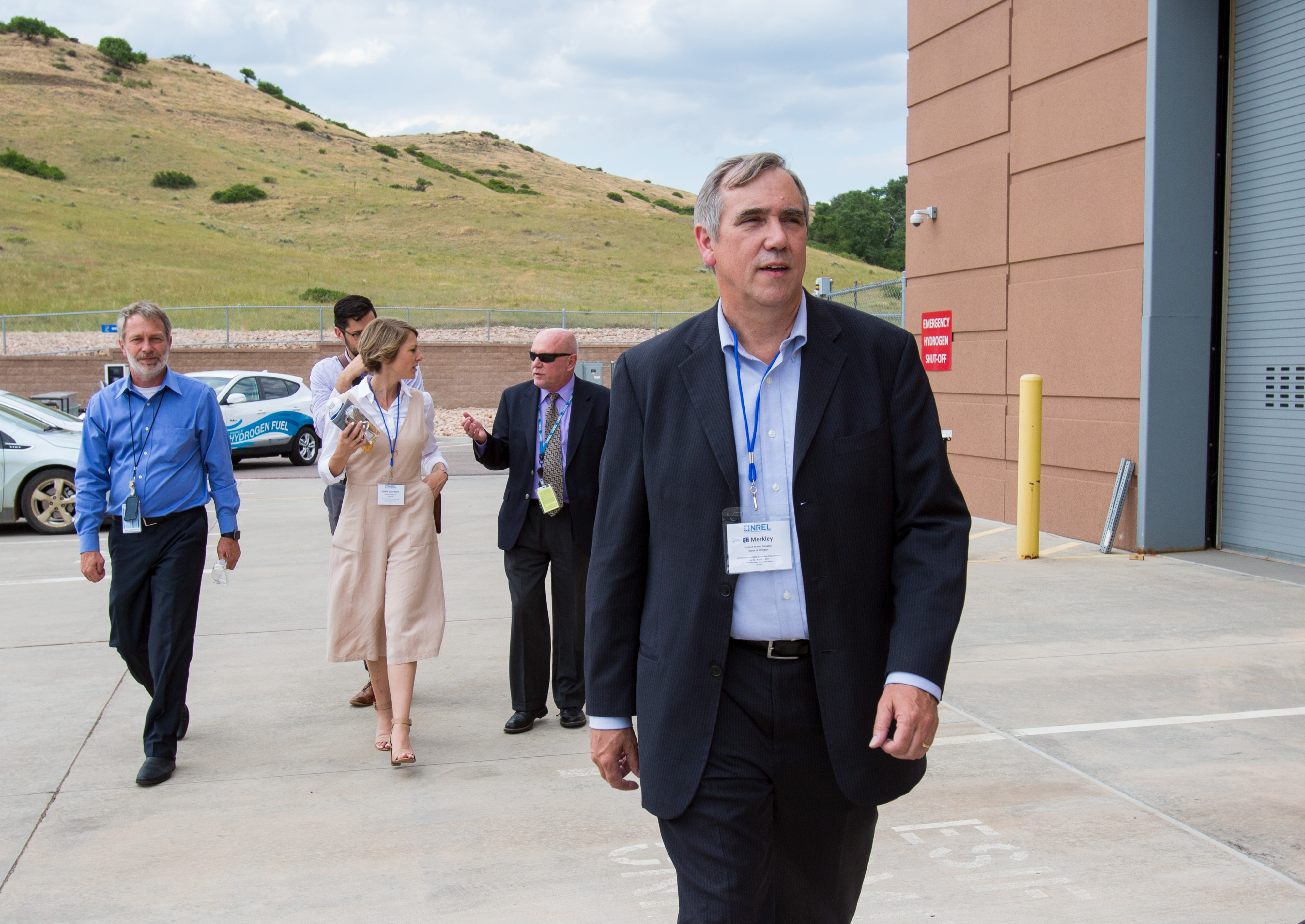This photograph captures a scene of five people walking near the back of a brown building, which has a large garage door and an emergency shut off sign. The main focus appears to be an older white gentleman, likely in his 50s or 60s, with gray hair that is longer on top and shorter on the sides. He is dressed in a navy blue suit jacket and matching pants, accessorized with a black leather belt and a wedding band. Underneath the jacket, he wears a light blue button-up collared shirt. A blue lanyard with an unreadable white pass hangs around his neck.

Accompanying him are four other individuals: three men and one woman. The men are dressed similarly in suits and ties, adhering to formal office attire. The woman stands out in her long-sleeved white blouse, tan-colored dress, and sandals, suggesting a warm climate. 

In the backdrop, there is a parking lot to the left with several parked cars, and a large green hill with trees behind a stone wall. This setting, together with the formal dress code, implies a professional environment situated in a somewhat industrial area, with a balance of nature visible in the background.